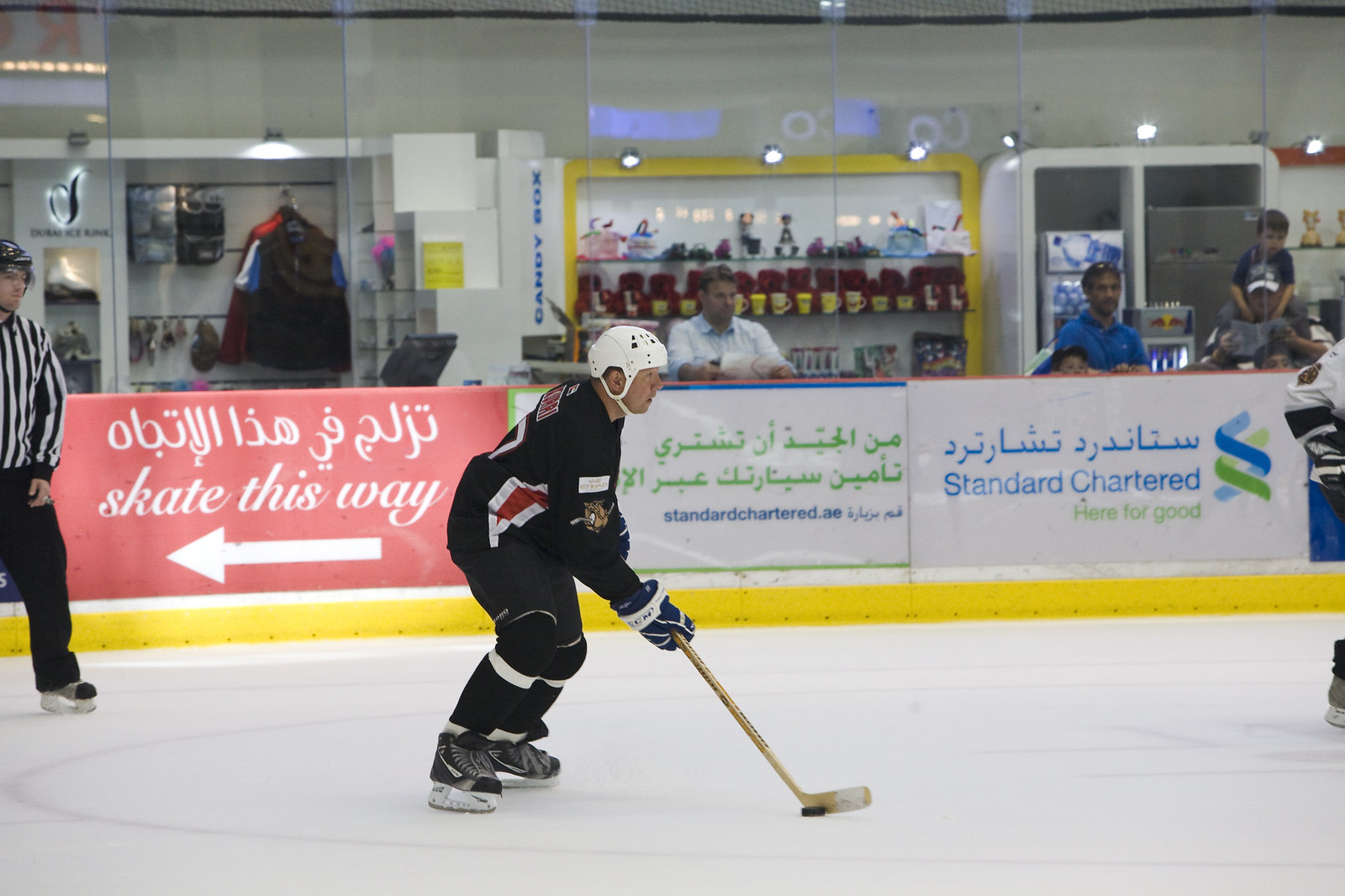The photograph captures an intense moment in an ice hockey game. At the center of the image is a focused ice hockey player in a black jersey with striking red stripes along the sides, black pants, and black ice skates with silver blades. He wears a white helmet with a strap under his chin and thick black mittens as he deftly controls a black puck with his light brown hockey stick, which has tape on the flat end. To his left, partially visible, is a referee dressed in black pants and a white and black striped shirt, overseeing the action on the white ice marked with various lines indicating different areas of play. On the right side, another player in a white jersey is just barely in the frame, their remaining attire indiscernible. The scene is set within a hockey arena, evidenced by the enclosed ice rink bordered by yellow-bottomed boards adorned with signs and advertisements in various languages, including English phrases like "skate this way" with an arrow and "standard chartered, here for good". Beyond the boards, spectators, including a man with a child on his shoulders, watch the game. The rink is polished and well-lit, with shiny surfaces reflecting the overhead lights, adding to the vibrant and dynamic atmosphere of the arena.